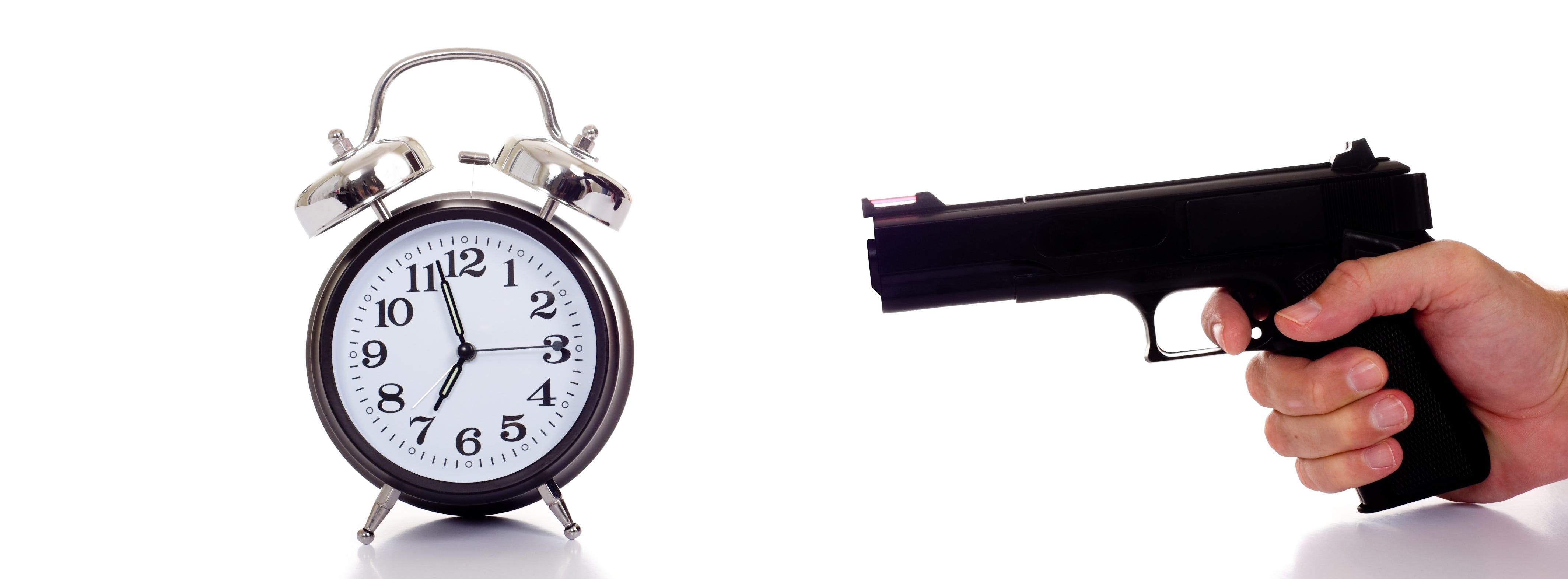In the image, a human hand is holding a black pistol, its finger on the trigger, aimed directly at an old-fashioned alarm clock. The background is pure white, casting only the shadows of the hand, gun, and alarm clock. The clock, located to the left of the gun, is a classic design with a black casing, white face, and black numbers, showing the time as approximately 6:57, almost 7 o'clock. The clock features two silver bells on top connected by a silver rod and has two silver feet at its base. The detailed elements of the gun and the clock, along with the stark simplicity of the white background, suggest a humorous portrayal of frustration with waking up early.